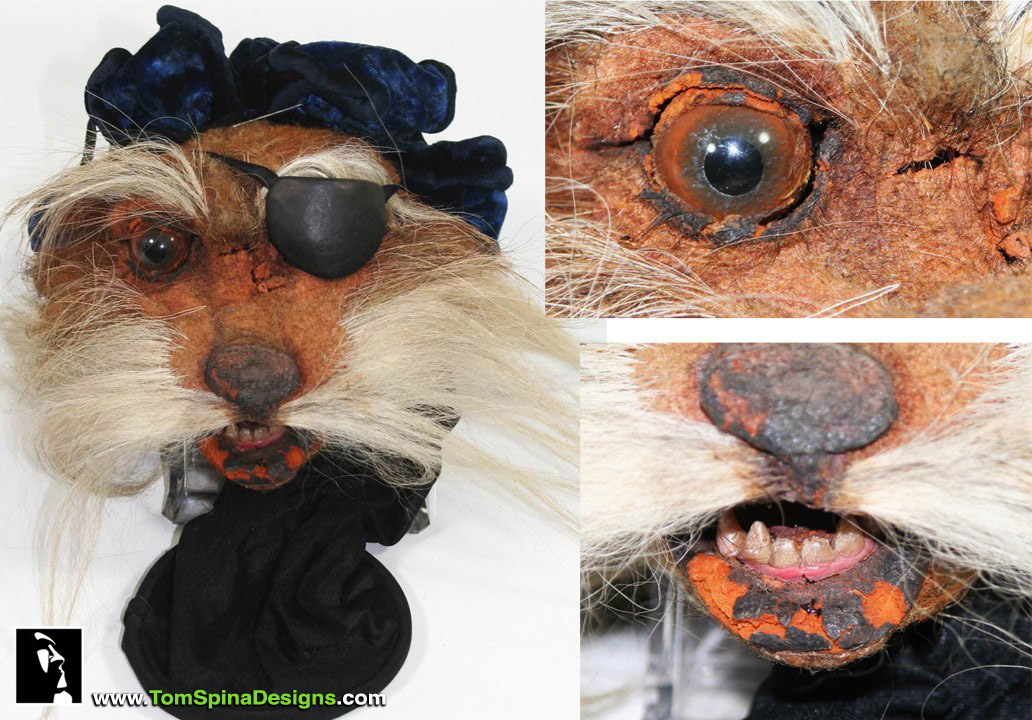The image showcases a deteriorating yet intricate fox-like puppet head, reminiscent of a movie prop, displayed in a set of three detailed photographs. The central image reveals the entire head, featuring gray hairs, with a large white mustache, and the skin visibly decayed and broken along the jaw, giving an appearance of falling apart. The puppet's bulging eyes stare straight ahead, one of which is covered with a black eyepatch. The fox-like creature dons a blue bonnet and has a black piece of fabric wrapped around its neck. The additional close-up photographs on the right provide more detail: the top image zooms in on an eye, displaying a large black pupil surrounded by various shades of gray and red, with a crusty red and black outer ring; the bottom close-up focuses on the mouth, highlighting the faded, aged yellowish teeth with surrounding deteriorated black and red crust. The background is a plain white, featuring the website www.tomspinadesigns.com at the bottom and a tiki head logo on the bottom left corner.